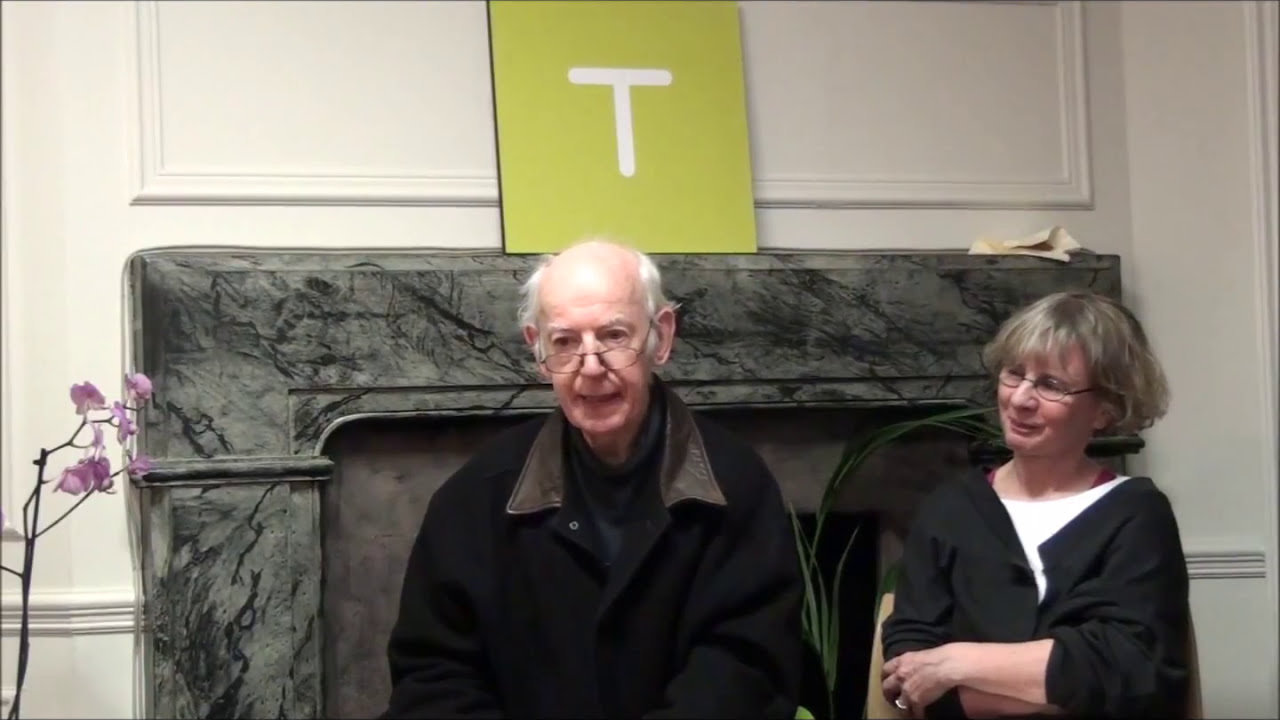The photograph is a rectangular indoor image capturing an older man and a slightly younger woman seated closely together, possibly indicating they are a couple. The man, likely in his 70s, is bald on top with gray hair on the sides, and is wearing glasses and sunglasses. He dons a black jacket with a leather collar over a navy blue turtleneck. His mouth is open, suggesting he is speaking. The woman to his right appears to be in her 50s, has dirty blonde, short silver-brown hair, and is also wearing glasses. She smiles at him while crossing her arms and holding her elbows. She is dressed in a white t-shirt with a black knit sweater or poncho over it. Behind them, a gray and black marble fireplace is visible, adorned with a lime green square sign displaying a large white capital "T." To the left of the fireplace mantle, an orchid with light purple and pink flowers is spotted. The background wall is white, adding to the indoor setting's brightness.